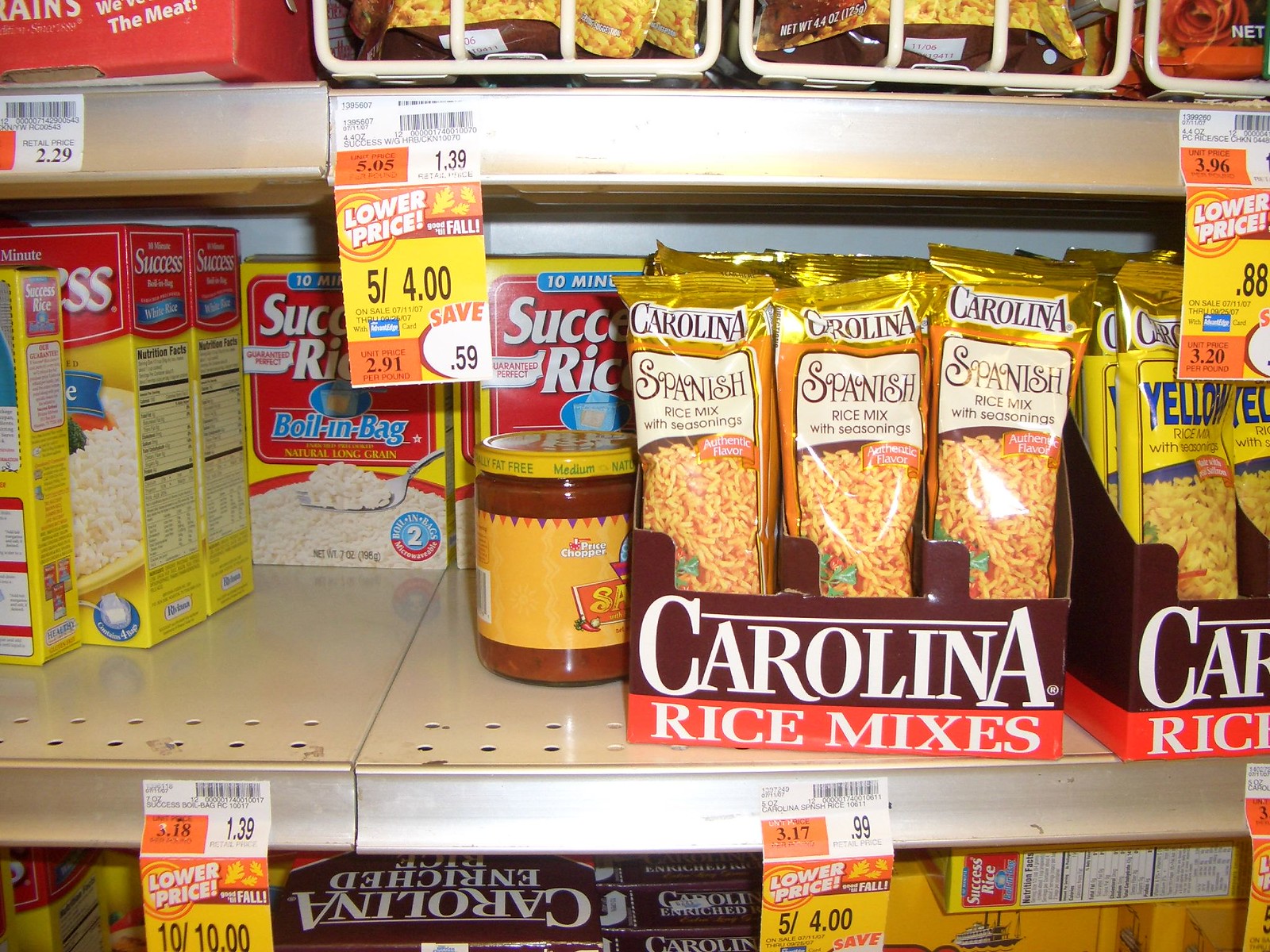In this image taken in a grocery store aisle, a middle row of a shelf is prominently featured. The shelf is stocked with various rice products, predominantly Carolina brand mixes. The central focus is on boxes containing Carolina Spanish Rice Mix with Seasoning, easily identifiable by their distinctive gold packaging. To the left of these boxes is a jar of salsa, positioned in front of two boxes of boil-in-bag white rice, which can be seen peeking from behind the salsa jar. Next to the salsa, there is a noticeable empty space, indicating a gap in the product display. To the far left of this empty space are more assorted rice packages, while to the right, additional boxes of Carolina Yellow Rice in golden bags are neatly arranged within a brown box. Dangling from the shelf are small, prominent price tags, one of which indicates a special deal: "Lower Price - 5 for $4." The well-organized yet varied assortment of products and price tags creates an engaging and realistic snapshot of a grocery store aisle.